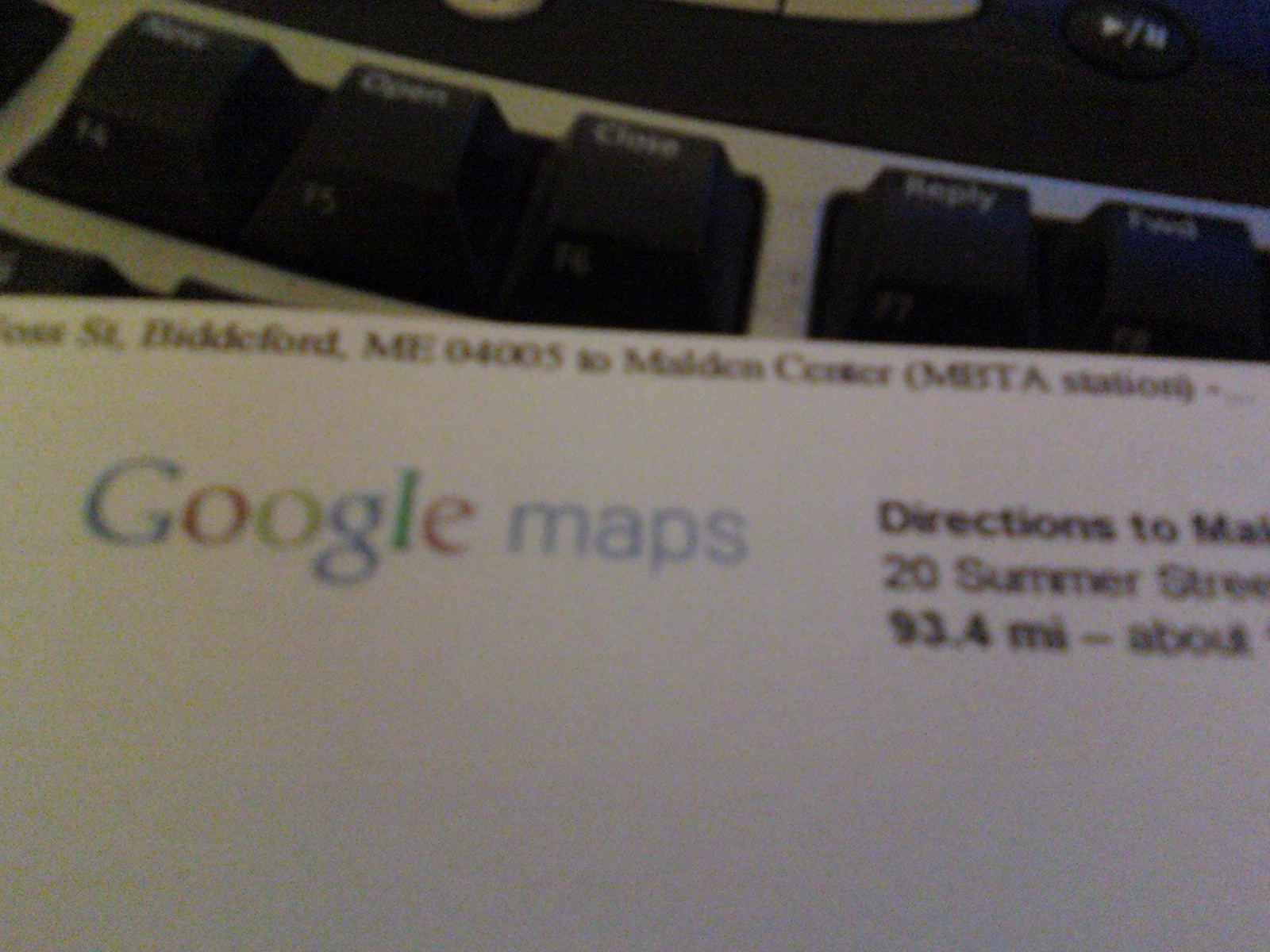A close-up blurry photo prominently features a section of a computer keyboard at the top. The keys displayed include "Open," "Close," and "Reply," all of which are small and black, though the key to the left of "Open" is indiscernible. Below the keyboard lies a printed sheet of paper carrying significant textual information.

Despite the blurriness, the top line of the paper seems to read: "something Street, Biddeford, ME 04005." The following line appears to mention "10 Maddon Center" or possibly "Madden Center" and includes the term "Station." These details are rendered in black text on a white background.

In contrast, a section of the paper features colorful text; "Google Maps" is displayed, with "Maps" in light blue. Below, the document provides directions to "20 Summer Street," estimated to be "93.4 miles - about."

The cohesive yet detailed description attempts to encapsulate the visual and textual elements present in the photo, despite its blurriness.